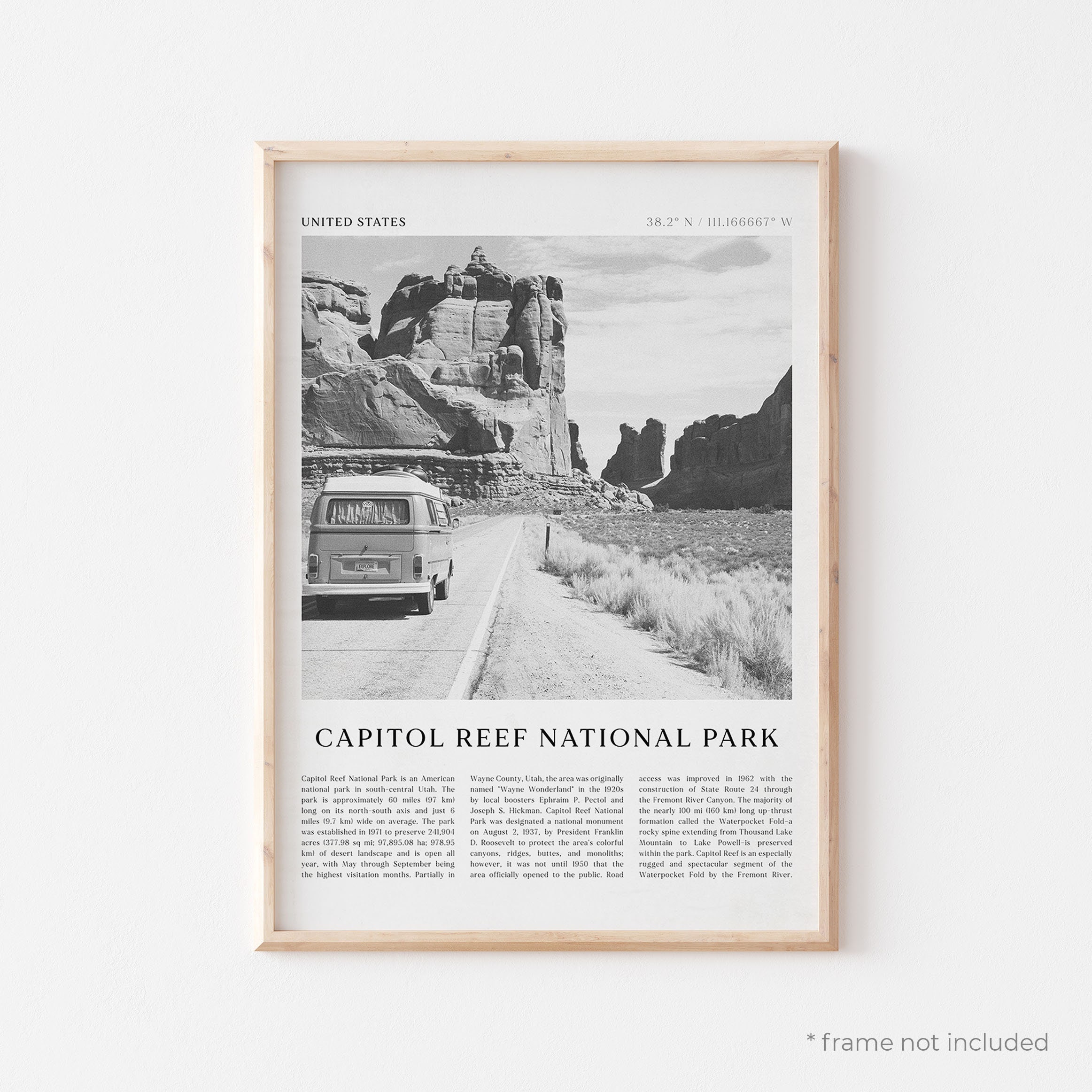This image is a black and white print framed in light brown wood, featuring a reprinted and enlarged article titled "Capitol Reef National Park." At the top of the article, the words "United States" are prominent alongside geographic coordinates: 38.2 degrees north, 111.1666667 degrees west. The main photograph displays a classic Volkswagen van traveling on a road towards striking rock formations typical of a desert landscape. On the right side of the image, small plants can be seen, adding to the natural scenery. Beneath the photograph, three columns of text provide details about Capitol Reef National Park. Additionally, a watermark on the bottom right corner clearly indicates that the "frame is not included," suggesting this might be an advertisement either for the image or for the frame itself.